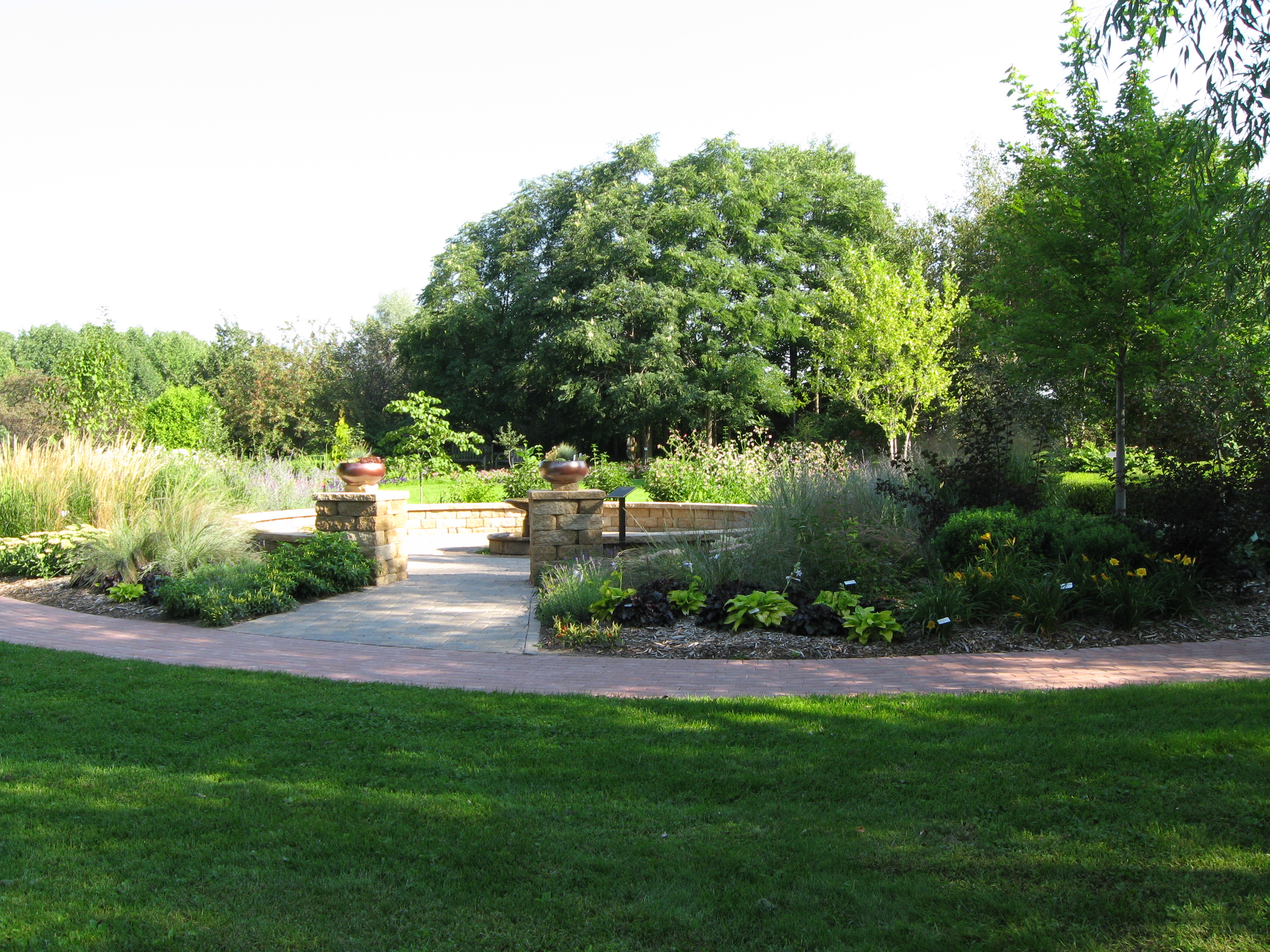A picturesque park area is showcased in the image, featuring meticulously trimmed grass that carpets the entire bottom portion in a vibrant green. A gently curved sidewalk, paved with red bricks, winds its way through the center, guiding the eye towards a charming garden rest area. This rest area is enclosed by a circular stone fence, accentuated by two sturdy stone pillars. Atop each pillar rests a brass bowl, adding a touch of classic elegance with their rich brown color.

In front of the fencing, a variety of shrubbery and flora burst forth in a riot of colors, including shades of green, light green, and hints of yellow from the blooming flowers. Amongst the lush greenery, a few tall, thriving trees stand proudly in the background, their leaves ranging from dark to light green, creating a vibrant canopy.

Peeking from behind the right stone pillar, part of a presumably brass fountain is visible, its corner matching the brown hue of the brass bowls. The fountain's partial appearance hints at its prominence within the garden, adding to the serene and inviting atmosphere of the setting.